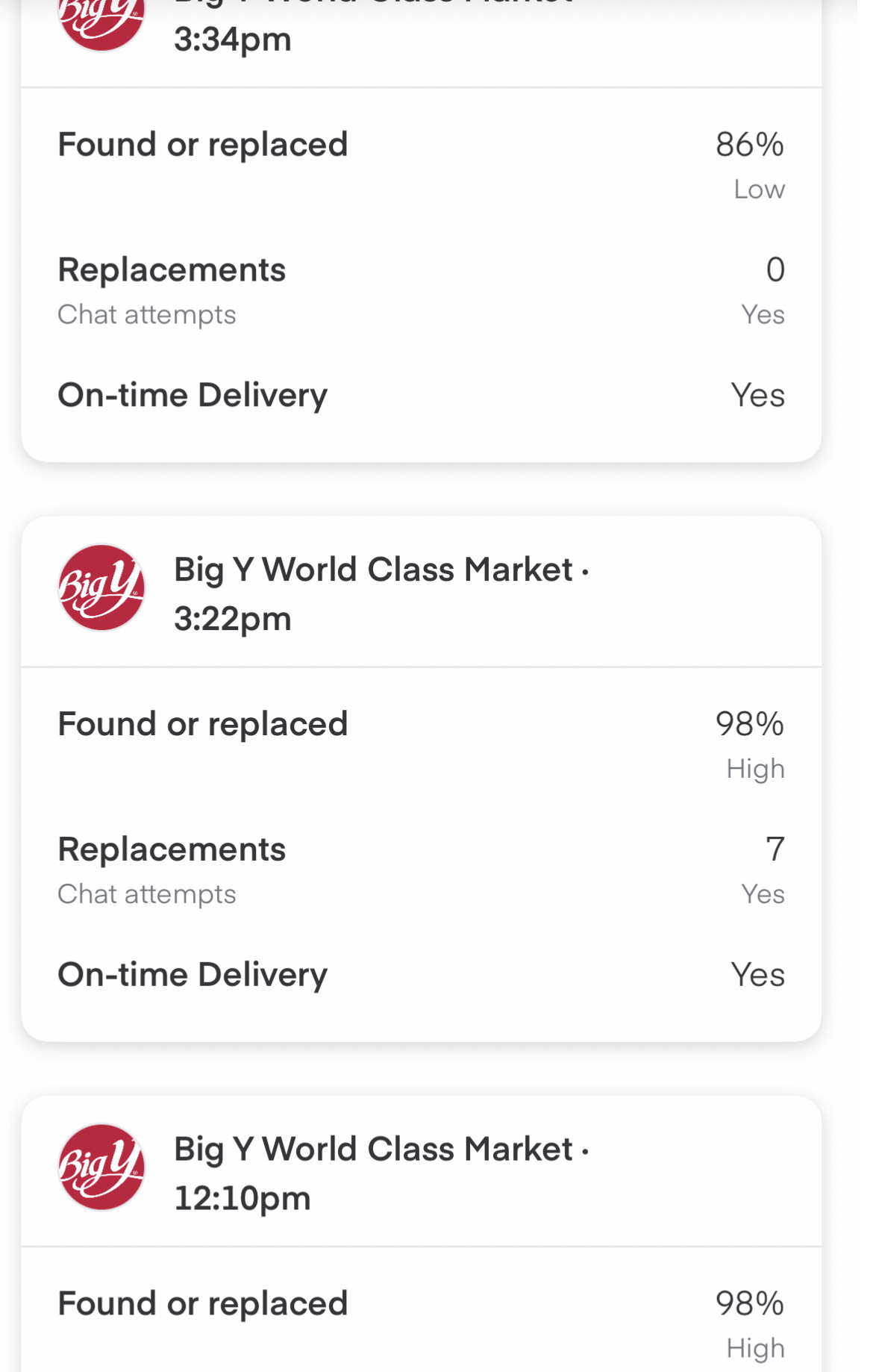This screenshot displays a vertical sequence of several neatly arranged items, each section presenting detailed information within a structured layout.

At the top of the screen, the first segment is partially cut off, with only the lower portion visible. It begins with the time stamp "3:34 pm" displayed prominently on a clean white background. Below this time stamp, a thin gray line serves as a divider, separating the time from the subsequent informational content arranged in three distinct rows. 

- The first row reads "Founder Replaced" with an 86% success rate, and underneath this indicator, the status is marked as "Low."
- The second row is labeled "Replacements," with a subtext that explains "Chat Attempts." To the right, it clarifies with "Zero" attempts and a "Yes" indicating a likely affirmative status.
- The third row states "On Time Delivery" with a confirming "Yes" to its right. Each of these informative rows is housed within a white rectangular box that is bordered by a light gray outline and features a subtle gray shadow, giving a sense of depth.

The next section follows the same structural format, starting with a distinct dark red logo featuring flowing white text that reads "Big Y" in the top left corner. Adjacent to this logo, black text spells out "Big Y World Class Market," accompanied by a black dot marker. Beneath this header, the time "3:22 pm" is indicated. Below, similar to the previous section:
- The first row displays "Founder Replaced" with a 98% success rate labeled as "High."
- The second row notes "Replacements," complemented by "Seven Chat Attempts," and a confirming "Yes."
- The third row mentions "On Time Delivery," also marked affirmatively with a "Yes."

The subsequent section further down the screen mirrors the preceding layout, although it is partially cut off at the bottom. The visible part shows the same red "Big Y" logo at the top left, followed by the "Big Y World Class Market" label and a dot marker, with the time "12:10 pm" noted beneath. Further listed details include:
- "Founder Replaced" again marked at 98% and categorized as "High."

The meticulously formatted sections on this screen provide a clear and organized presentation of various metrics, statuses, and timestamps, each set against a white background with light gray accents contributing to a professional and polished appearance.